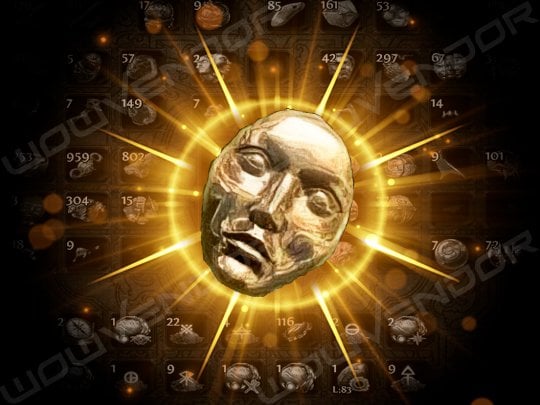The digital artwork showcases a central stone face mask, slightly bronzed with metallic hues, lying on a surface and looking directly at the viewer. Behind the mask, a radiant golden ring resembling the sun emits glowing, spiked rays that stretch outward. The image is set against a dark background filled with numerous semi-transparent squares, each containing indistinct icons, possibly of animals or other masks, and numbers varying from 1 up to the 900s in the upper left corners. A barely readable, diagonal watermark inscribed with "W-W-V-E-N-D-O-R" overlays the background, further adding to the intricate and enigmatic nature of the piece.